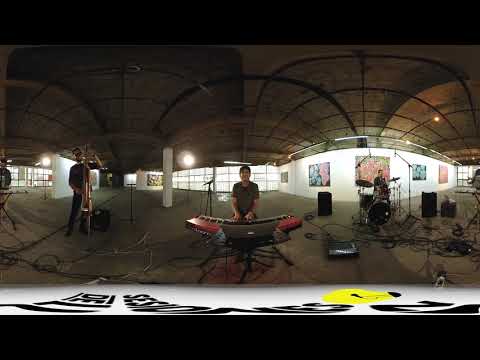This image captures a dynamic indoor scene of a band playing music in what appears to be an empty warehouse or an art gallery. The setting is industrial, characterized by a wooden ceiling with support beams, white walls adorned with brightly colored, abstract artwork, and large windows letting in natural or artificial light. The image has a slight distortion, suggesting it may be a 360-degree panoramic shot. 

At the center of the photograph, a man, likely Caucasian and wearing a short-sleeved shirt, is playing a red and black keyboard. To his right, a drummer is positioned with a complete drum set. To the left of the keyboard player stands a tall man in a black shirt, playing a gold woodwind instrument, possibly a saxophone. The floor is a hard surface, possibly concrete, cluttered with numerous wires, speakers, and other musical equipment, creating a hectic but artistic and authentic atmosphere. The top and bottom of the image are bordered by a solid black strip, with an unreadable banner just above the bottom border. The image is richly detailed with colors including black, white, yellow, red, gray, pink, purple, light blue, and orange, emphasizing the vibrant and eclectic feel of the scene.